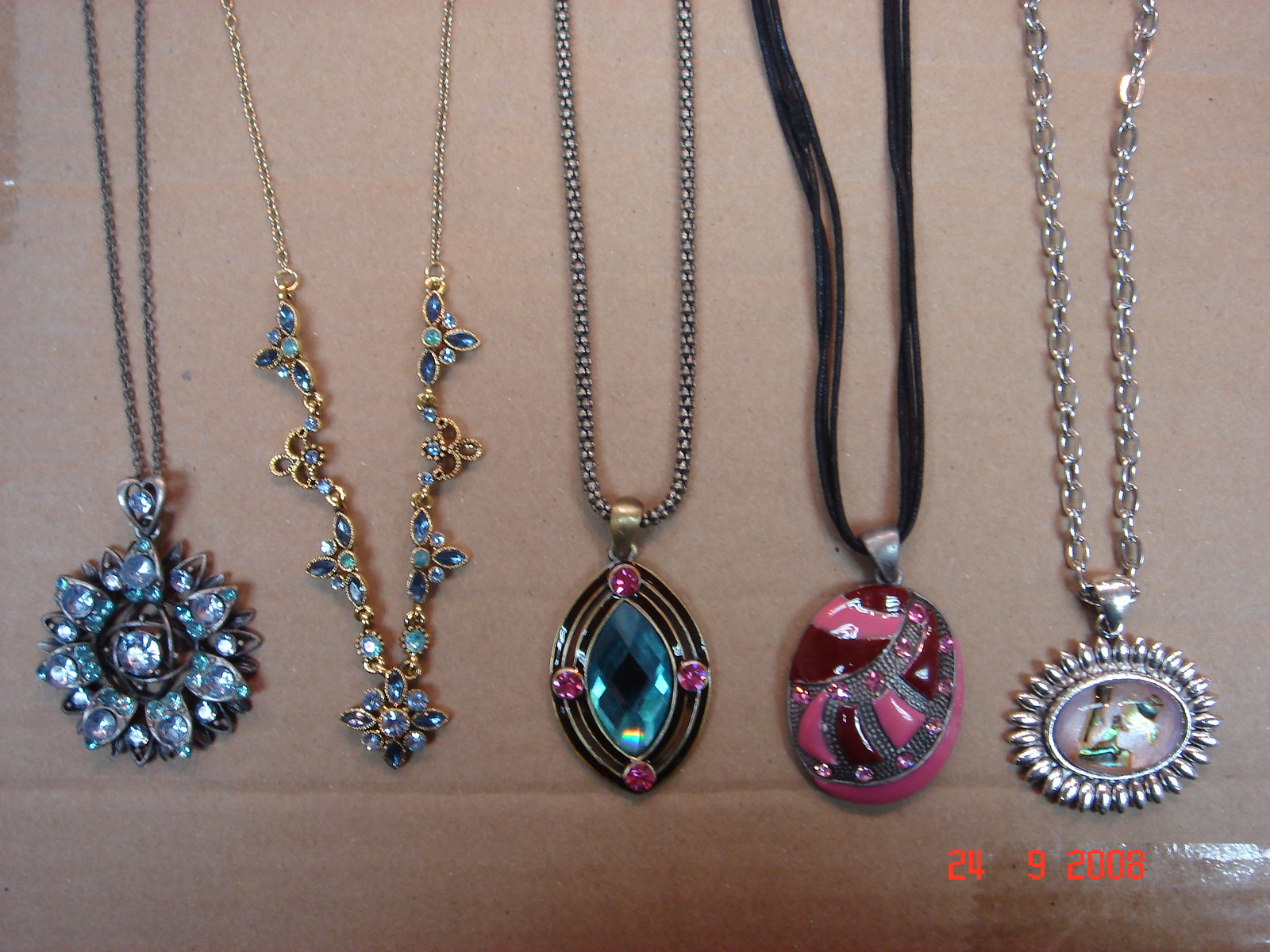This is a photograph of five intricately designed necklaces displayed horizontally on a grayish beige, possibly cardboard background. A small piece of clear cellophane tape with the red date "24-09-2008" is visible in the lower right corner, indicating the photo was likely taken indoors.

1. The first necklace, on the left, features a metal silver chain and a pendant resembling a snowflake, adorned with blue stones in a floral design.
2. The second necklace has a gold chain lined with alternating blue and gold floral designs, ending in a larger blue gemstone.
3. The third necklace, which seems to have a gray or possibly a thicker silver chain, boasts an oval-shaped pendant with a central blue stone surrounded by purple stones.
4. The fourth necklace, supported by a black leather or faux leather strap, sports a mixed-color pendant featuring shades of purple and pink in a swirling pattern.
5. The final necklace on the right has a gold interlinked chain with a pendant that includes a purple center stone encased in a silver border.

These elegant pieces are laid out flat, with their pendants prominently displayed, showcasing the variety of designs and colors in a visually appealing arrangement.